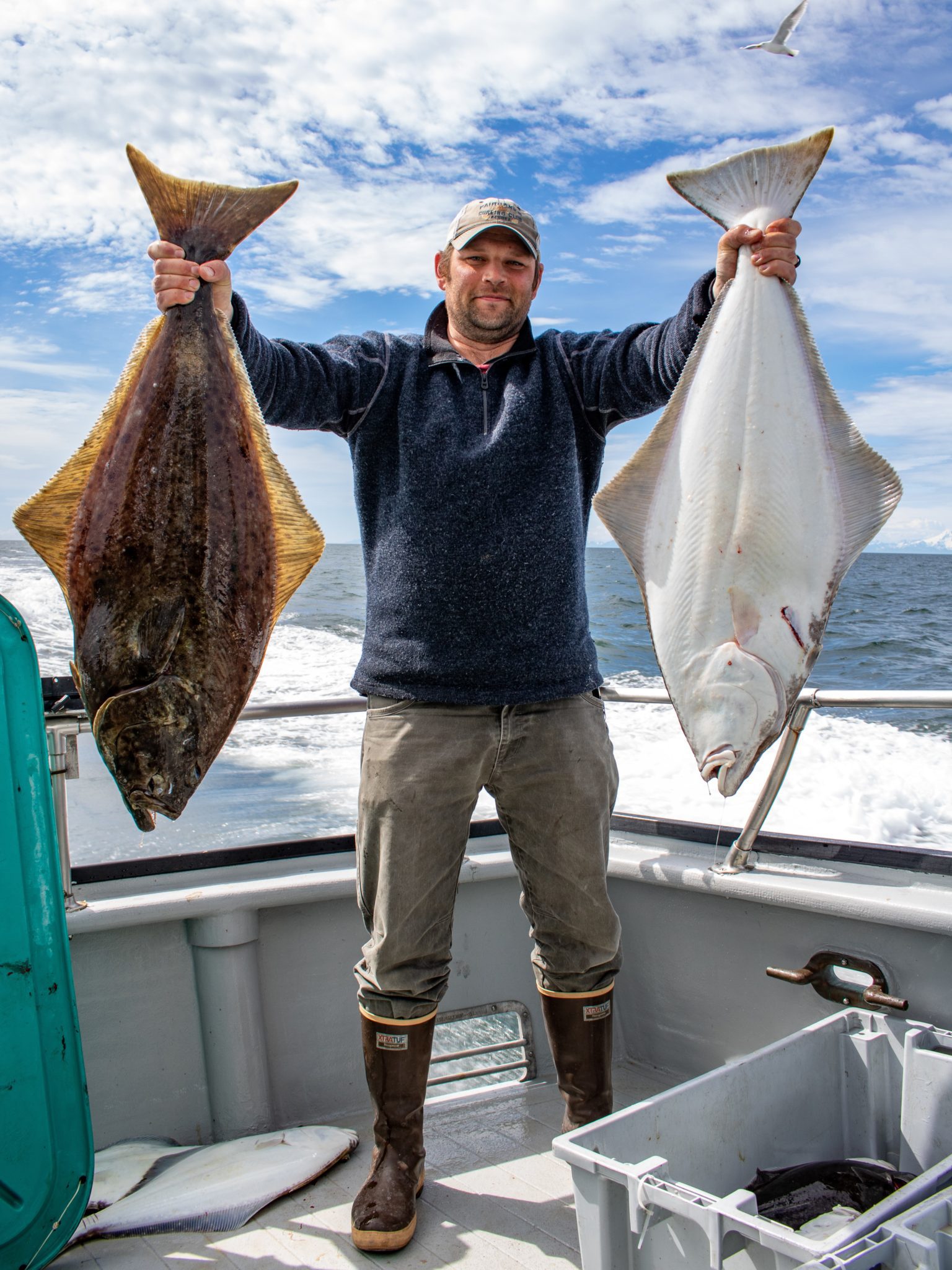In this vivid color photograph, a fisherman stands at the rear of a motorboat, moving swiftly across the blue ocean, as evidenced by the trail of white churned up by the boat's motor. The sky above is blue with scattered clouds, and a seagull can be seen soaring overhead. The man, clad in a green baseball cap, a blue long-sleeved half-zip pullover, faded blue jeans, and green fishing waders or boots, proudly holds up two very large fish. Each fish, approximately half the length of the man's body, has a triangular shape with fins extended. The fish in his right hand is white, likely displaying its belly, while the one in his left hand is a dark gray-brown. The boat's gray interior contains various gear, including a gray tackle box in the foreground and a large tub near the man, possibly holding smaller fish. Additionally, two smaller fish, similar to the ones he is holding, lie on the deck to his right.